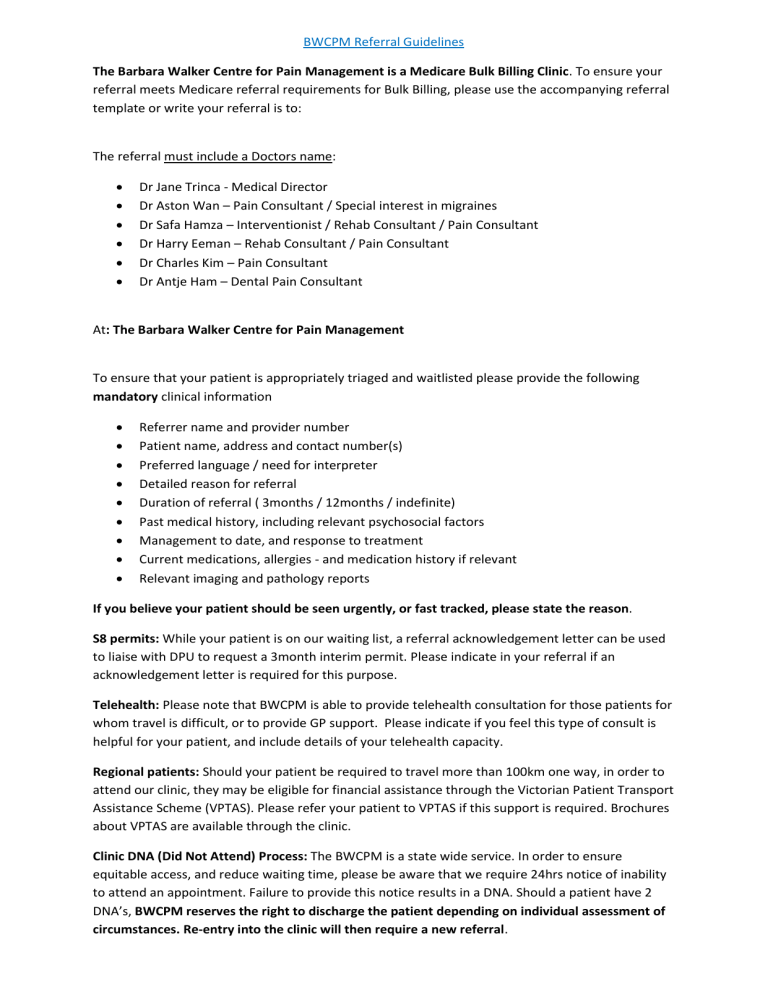The image appears to be a document, primarily white with extensive black text. At the top center, it features blue, underlined text that reads "BWCPM Referral Guidelines." Below this heading is bolded text stating, "The Barbara Walker Center for Pain Management is a Medicare bulk billing clinic," followed by a detailed description.

Three lines underneath, bold text informs that "the referral must include a doctor's name," and then lists seven bullet points with names of doctors such as Dr. Jane Trinca, Medical Director, and Dr. Aston Juan, Pain Consultant, among others.

Further down, another section in bold reads, "At the Barbara Walker Center for Pain Management," followed by more bullet points detailing mandatory clinical information required for proper triage and waitlisting of patients. These points include:
- Referring doctor's name
- Provider number
- Patient name
- Preferred language
- Detailed reason for referral
- Duration of current condition
- Past medical history and management to date
- Current medication
- Relevant imaging and pathology reports

Next, there are five paragraphs of text, each beginning with bolded headings:
1. "If you believe your patient should be seen urgently or faster, please state the reason."
2. "S8 permits," followed by a detailed description.
3. "Telehealth," with additional explanatory text.
4. "Regional patients," and further details.
5. "Clinic DNA (Did Not Attend) process," with more text.

At the very bottom, bold text reads, "BWCPM reserves the right to discharge the patient depending on individual assessment of circumstances. Re-entry into the clinic will then require a new referral."